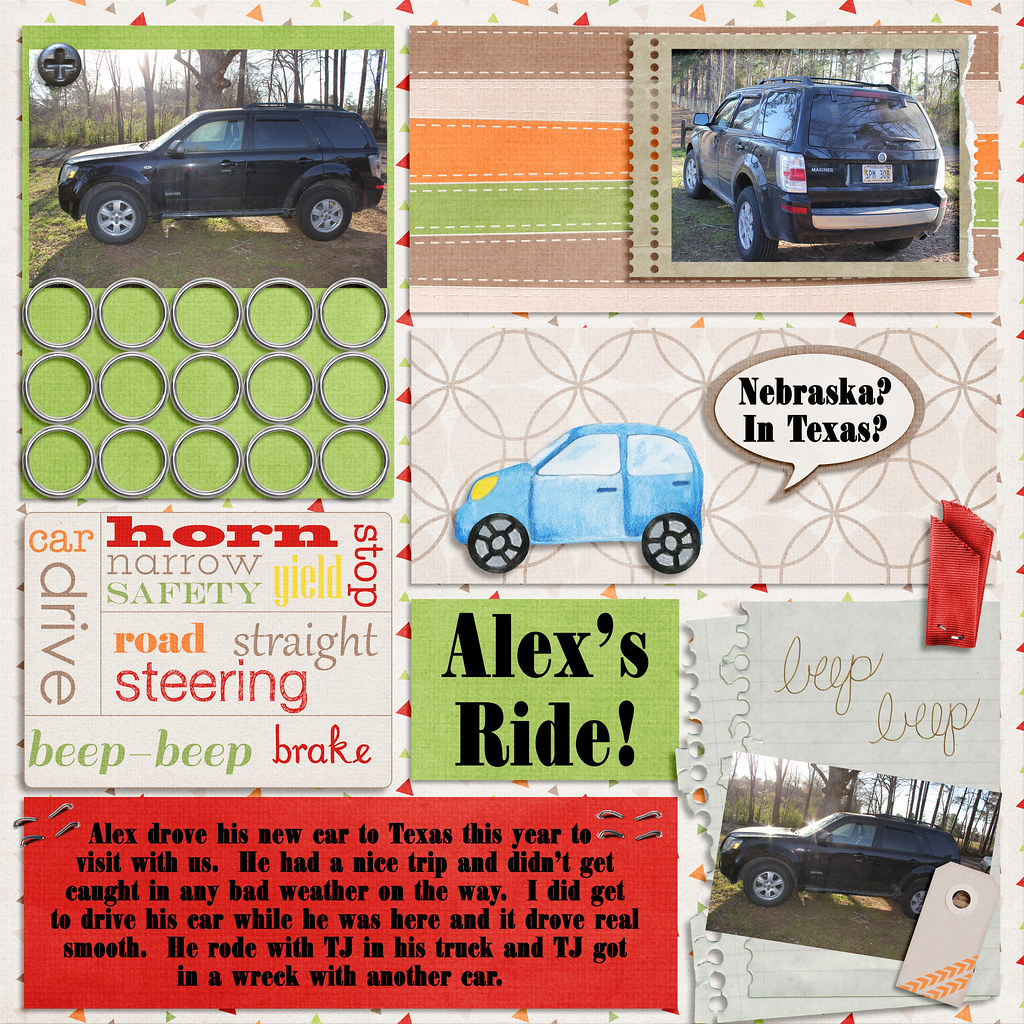This poster-flyer hybrid showcases a vibrant, square design brimming with visual elements and text against a light background adorned with festive confetti or colored triangle patterns. 

In the upper left corner sits a photograph of a black SUV facing left, bordered by a green frame. Beneath this SUV image are three rows of metallic silver rings, followed by a white box filled with various automotive terms like "road," "steering," "straight," "beep," and "brake." Adjacent to this section, occupying the middle to right part of the poster, are horizontal stripes in brown, white, orange, green, and gray hues, beside which is another image of the SUV, this time viewed from behind and angled to the left.

Below this image, a cartoonish blue car driving leftward features speech bubbles exclaiming “Nebraska?” and “Texas?”. Directly underneath this illustration lies a small green box with "Alex's Ride" inscribed in black letters.

Towards the lower left of the poster, extending towards the middle, a red rectangle contains six lines of black text. Meanwhile, the overall composition includes scattered words like "horn," "narrow," "safety," and "stop" in whimsical, multicolored fonts.

Lastly, the bottom right corner displays a sketch-like representation of a black SUV facing left on what appears to be sheets of paper, with the word "beep" inscribed above it. This section is marked by a small, red fabric piece at the top right and a tag extending from the bottom, covering part of the SUV's rear.